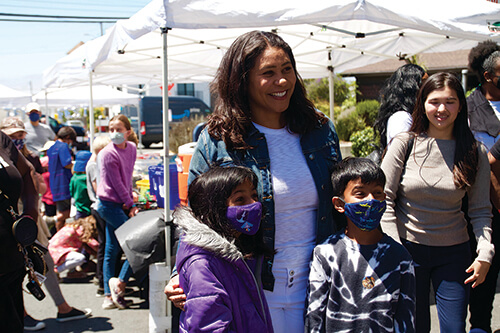The photograph, taken at an outdoor fair or farmer's market, captures a central scene with a woman of dark complexion and long black hair. She is wearing a white top paired with white jeans and a blue denim jacket, and is smiling with apparent joy. Flanking her, she has her arms around two children, likely her own. On the left, her son, dressed in a black and white tie-dye or striped long-sleeved shirt and a blue COVID mask, stands close. On the right, her daughter, wearing a purple coat along with a matching purple COVID mask, is at her side.

In the immediate background to the right, a woman in a tan top with dark brown hair walks towards the camera, seemingly unaware of being photographed. Beyond her, the scene is bustling with activity under several white freestanding tents, characteristic of a farmer's market or similar event. Visible beneath one tent, there's a Gatorade-style canister on a table, and many attendees are seen wearing facial masks. The backdrop features some plants or bushes, and a parking lot with various trucks, including an identifiable Amazon Prime truck. The sky above is a clear blue, enhancing the vibrant outdoor ambiance.